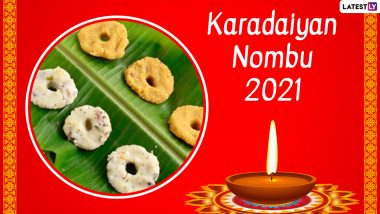The image appears to be from a food item label and features a bright red-orange rectangular background with vertical brocade-type yellow stripes on either side. In the upper right corner, there is a small mark that reads "latest" followed by someone’s initials. 

Dominating the left half of the rectangle, there is a large white-rimmed circle containing a photographic image. This image shows a banana leaf holding six ring-shaped confections that resemble pineapple rings or cookies, with three of them being tan and three white in color, all with a slightly lumpy texture. These items are laid out on a green placemat or a satin background.

In the bottom right section of the rectangle, there is a shallow dish containing a lit oil candle, placed on a trivet. The text on the label reads "Kara Daian Nombu 2021," suggesting the name and perhaps the year of the product or event being advertised.